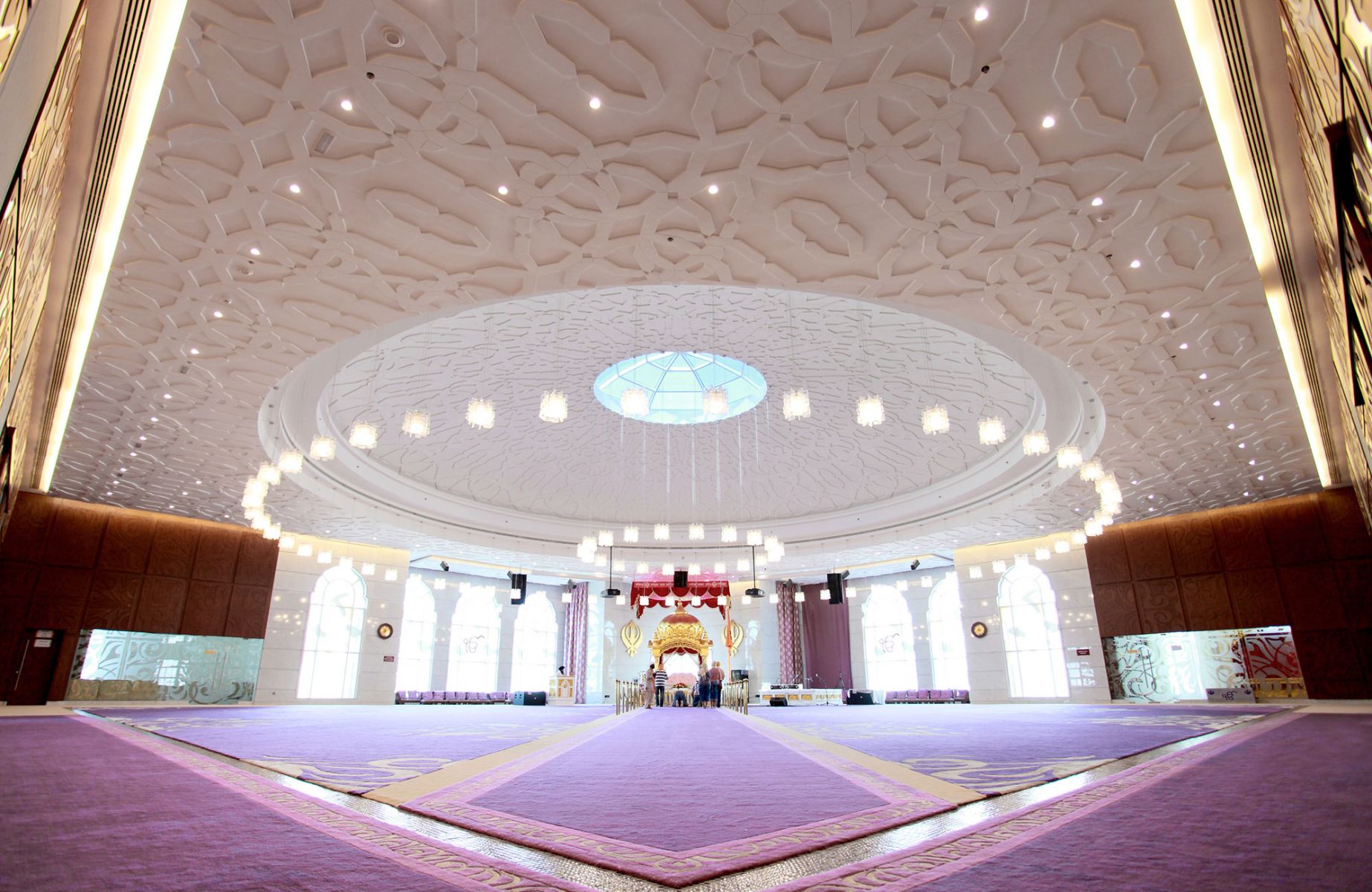A stunning photograph captures the grand entrance of a majestic historical building or luxurious hotel, featuring a vast and opulent interior. The focal point is a magnificent circular dome ceiling that commands attention. Nestled within the recess of this dome is a small, intricately-designed circular window composed of numerous panels, allowing a cascade of natural light to filter into the room. Below, the expansive room is adorned with plush purple carpeting that provides an opulent contrast to the surrounding architecture.

Lining the back walls are towering cathedral windows that infuse the space with a sense of grandeur and elegance. At the heart of the room stands a grand entranceway, resplendent with golden crown moldings that highlight its regal significance. In the foreground, a line of people wait patiently, adding a human element that underscores the building's significance as a place of interest or gathering. The overall ambiance and detailed craftsmanship conjure an exotic, palatial allure reminiscent of iconic structures like the Taj Mahal.